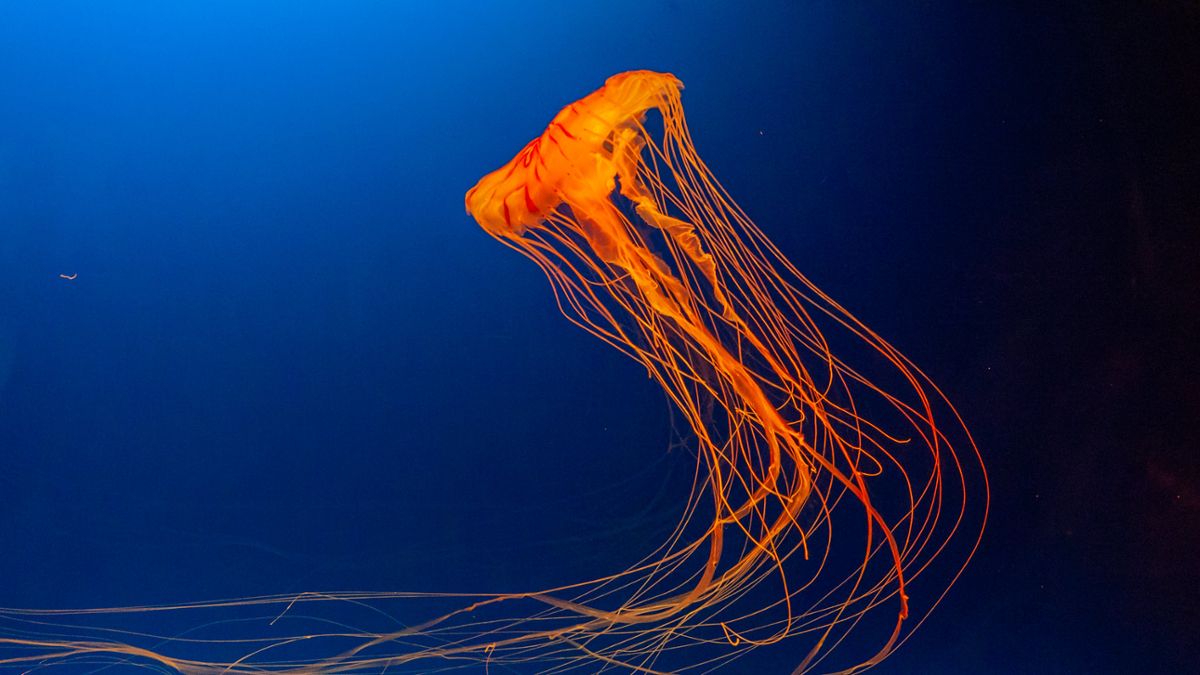This image captures a vibrant, striking photograph of an orange jellyfish with a flat, wavy head, resembling a stool. The jellyfish features a radiant mix of orange and red hues, particularly concentrated at the top of its head. Numerous thin, orange streamer-like tentacles, akin to roots, extend and curve gracefully to the left. These tentacles, notorious for their painful sting, add to the creature's mesmerizing appearance. The backdrop is a gradient of deep ocean blues, transitioning from a dark blue on the right to a bright, electric blue on the left. Specks of unidentified particles are scattered throughout the clear blue water, suggesting a natural, underwater setting. The photograph’s vibrancy and lack of other sea creatures or features evoke a sense of depth and isolation, making the jellyfish the focal point of this stunning and possibly enhanced underwater scene.